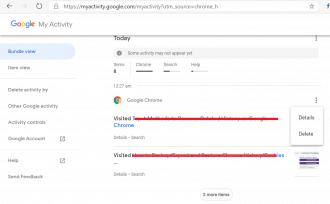This screenshot is taken from the "Google My Activity" page, displaying a summary of recent activity. "Google" is prominently displayed at the top in multicolored lettering (blue, red, yellow, blue, green, red). On the left-hand side, there is a vertical menu listing options such as "Bundle View," "Similar Google Activity," "Activity Controls," "Google Assistant," "Help," and "Send Feedback," though some of the text is too blurry to read clearly. 

On the right-hand side, there's a heading that reads "Today" with a note indicating that some recent activity may not yet be displayed. Below, the activity log records an entry from "12:27 AM" stating "Google Chrome, Visited," followed by a red-crossed line. Another line mentions "Chrome, Detail Search" with options for "Details" and "Delete," also crossed out in red. A small oblong icon is present at the bottom of the screenshot, but it is too blurry to decipher. 

The screenshot is devoid of any photographic elements, people, animals, birds, or plant life. The image solely focuses on the textual and interface elements of the "Google My Activity" page.